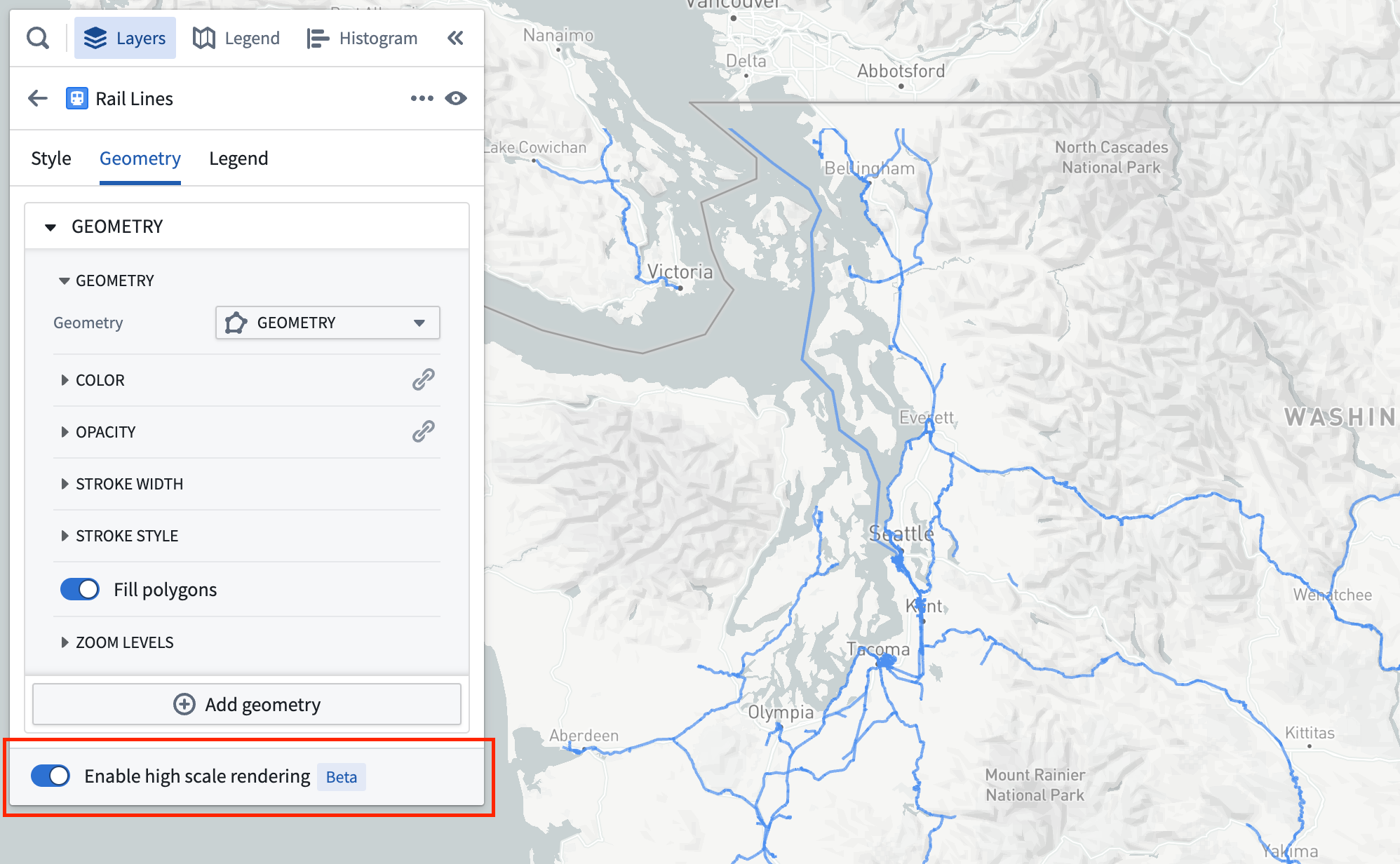This detailed digital map of Iowa showcases the state's layout with its major cities clearly marked, including Des Moines, Indianola, Ottawa, Kirksville, and Madison. The map interface is equipped with a variety of functional buttons and tools such as Layers, Find, Histogram, and Info for enhanced navigation and data analysis. An 'Add to Map' button with a plus sign allows users to incorporate additional elements into the map.

There's also a comprehensive styling menu featuring options like Save Styles, Default Styling, Rail Lines, and the Map Box Light theme. A pop-up window regarding Geometry includes adjustable options for Color, Opacity, Stroke Width, and Stroke Style. The currently selected Field Polygons are evident, although the 'Include in Legend' option is not activated.

Additional features include an 'Add Styler' button, as well as Label and Tooltip functionalities for further customization. Notably, the 'Enable High Scale Rendering Beta' option is selected and highlighted in red, indicating advanced rendering capabilities for detailed map visualization.